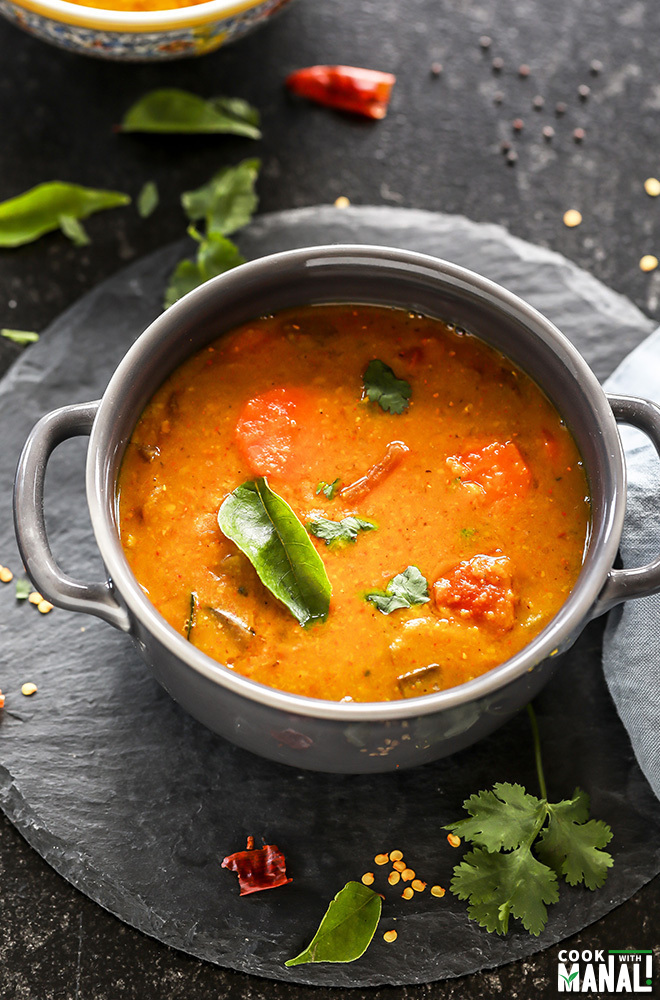In this vibrant and detailed photograph, we see a culinary masterpiece artfully composed on a black stone table. Central to the image is a circular stone plate of a dark, almost black hue, which seems carved from the same material as the table itself. Atop this plate sits an individual soup crock, crafted from gray ceramic and adorned with delicate handles on each side. This crock contains a rich, orange tomato-style soup that is thick in consistency, reminiscent of a hearty chowder. The soup is garnished with sprigs of green leaves, possibly cilantro or parsley, and scattered with red pepper flakes and peppercorns.

Surrounding the crock, on the edges of the plate, are more decorative arrangements of green leaves, seeds, and pieces of red pepper, adding bursts of color and texture to the earthy tones of the stone and ceramic. The scene is meticulously detailed, with each element thoughtfully placed to enhance the visual appeal of the dish.

In the bottom right-hand corner of the image, the words "Cook with Manal!" are printed in a clean white script, inviting viewers to join in the culinary journey. This logo adds a final touch of personality and branding to the photograph, capturing the essence of a well-crafted and appetizing presentation.